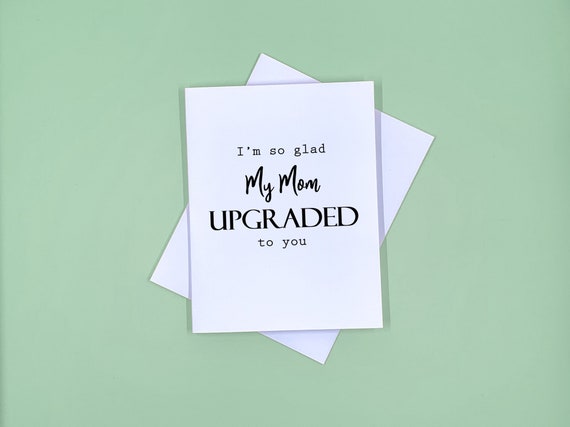The image features a computer-generated greeting card set against a green background. The card, which is predominantly white, is placed on top of a slightly angled white envelope but remains centered. The card bears the message, "I'm so glad my mom upgraded to you." This text is crafted using three distinct fonts: "I'm so glad" and "to you" in one font, "my mom" in a cursive style, and "upgraded" in an uppercase, arial-like font. All the text is in black, adding contrast against the white card. The scene contains no other objects, making the simple yet detailed design of the card the focal point of the image.